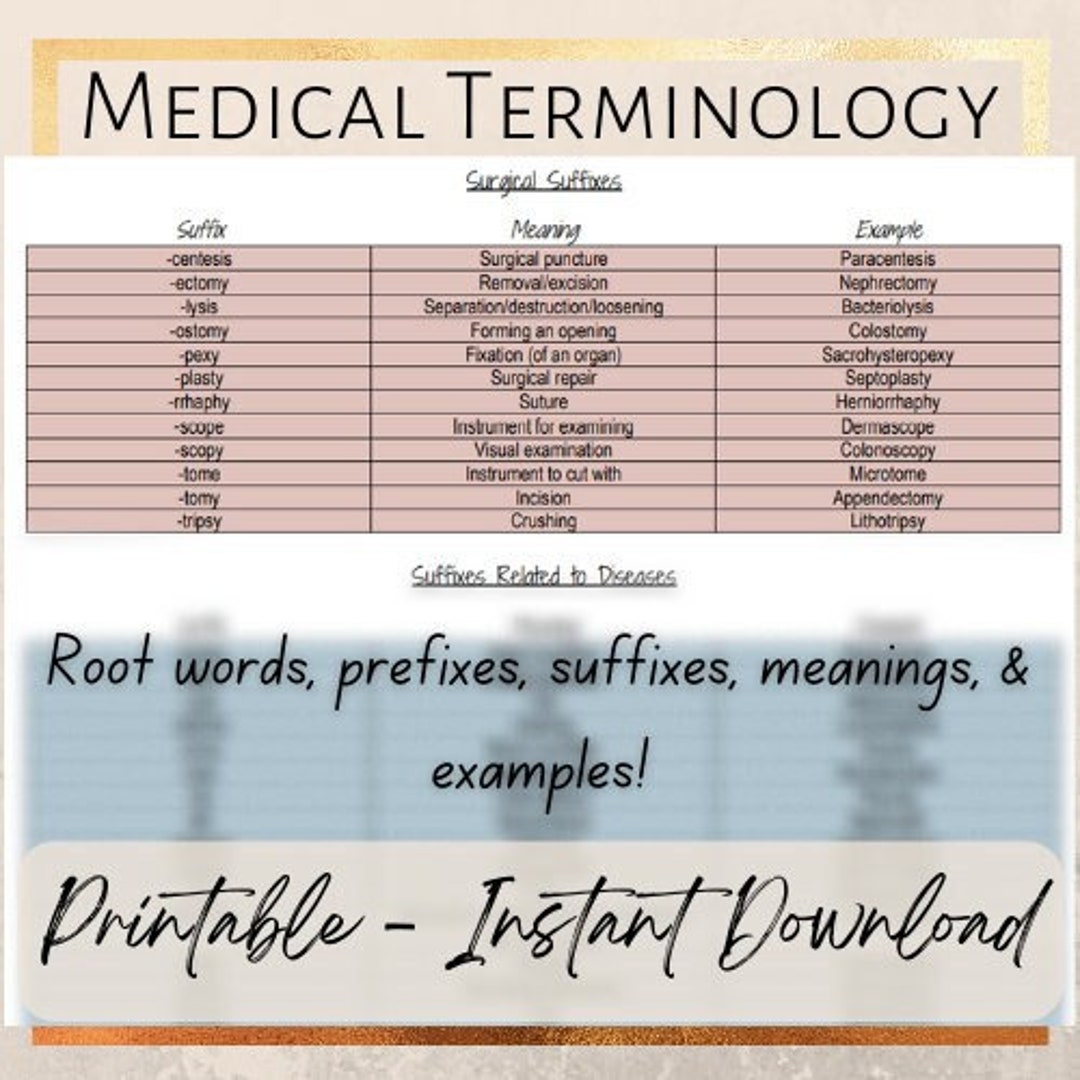This image is a detailed chart for medical terminology, primarily designed for educational purposes, possibly aimed at medical students or professionals. The top of the chart features the title "Medical Terminology" against a tan background. Below this, in a section with a white background, it lists "Surgical Suffixes." The chart itself is organized into three columns with multiple rows. The first column, in italics, lists various surgical suffixes such as -centesis, -ectomy, -lysis, -ostomy, -pexy, -plasty, -rrhaphy, -scope, -scopy, -tome, -tomy, and -tripsy. The second column provides the meanings of these suffixes, including terms like surgical puncture, removal/excision, separation/destruction/loosening, forming an opening, fixation (of an organ), surgical repair, suture, instrument for examining, visual examination, instrument to cut with, incision, and crushing. The third column gives examples of words that use these suffixes, such as paracentesis, nephrectomy, bacteriolysis, colostomy, sacropexy, septoplasty, herniorrhaphy, dermatoscope, colonoscopy, microtome, appendectomy, and lithotripsy.

Additionally, below the surgical suffixes section, the chart continues with "Suffixes Related to Diseases," followed by sections detailing "Root Words," "Prefixes," "Suffixes," "Meanings," and "Examples." The entire chart is designed in a visually organized manner, with black lettering against alternating backgrounds of blue and purple. At the bottom, it mentions that the chart is available as a printable, instant download, suggesting its availability for virtual access and easy printing.